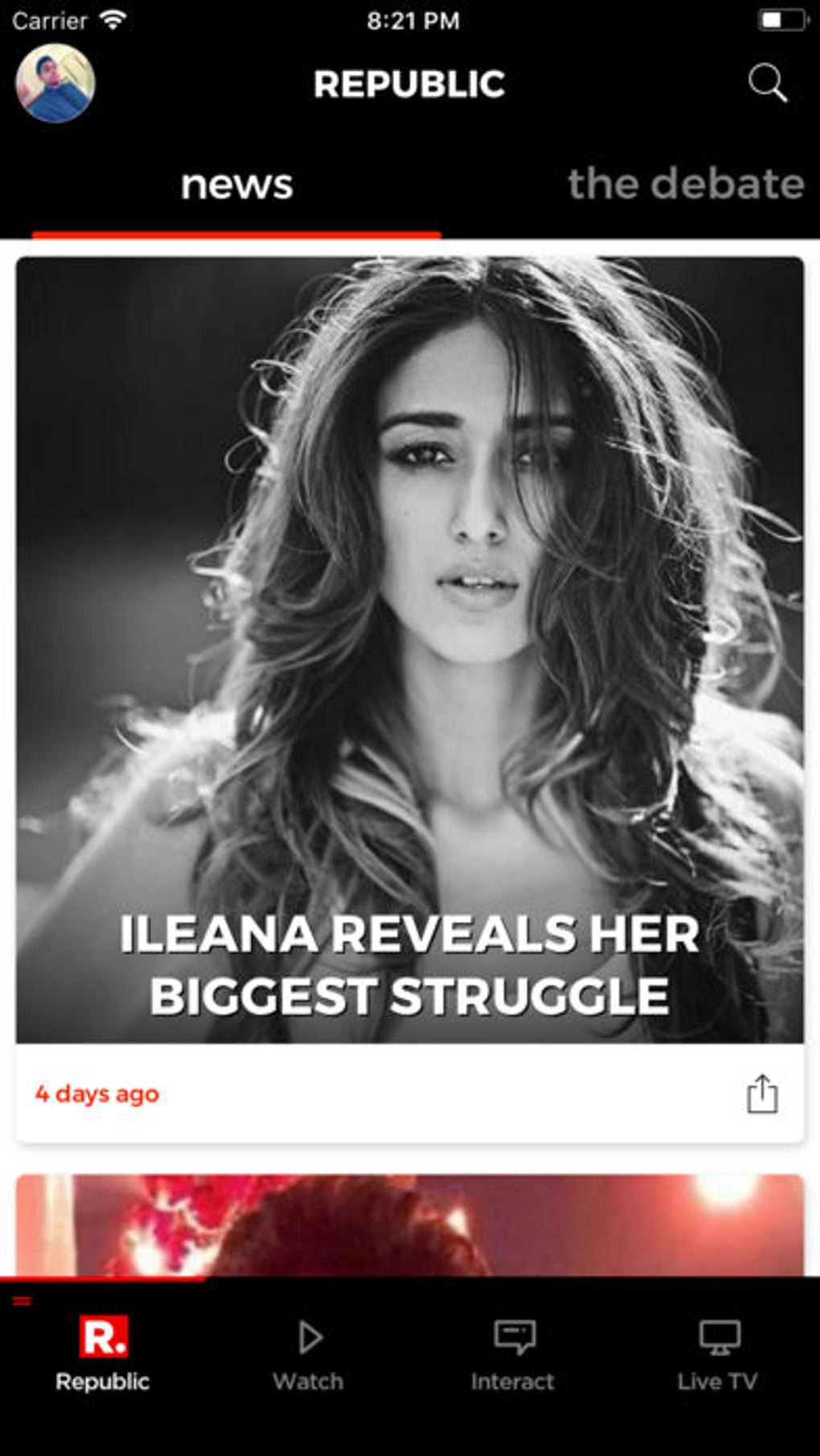The image is a vertically rectangular screenshot taken from a cell phone. At the top of the screen, there is a black horizontal banner displaying the carrier name on the upper left, next to a Wi-Fi icon. Directly below that, a circular avatar of a person can be seen, although details are indistinct, showing only a blue shirt and black hair. Centered at the top, the current time is clearly marked as 8:21 PM. 

Underneath the time, in bold, uppercase letters, the word "REPUBLIC" is prominently displayed. Directly below this, the interface offers two side-by-side options labeled "NEWS" and "DATE." The main content section features a white background with a black and white photograph of a woman with very long hair. At the bottom of this image, text reads, "Ileana reveals her biggest struggle." Just below this photograph, on the bottom left corner, it indicates that the story was published four days ago. The very top portion of another image is visible beneath the main photo, hinting at the continuation of additional content. 

The bottom of the screenshot features another black horizontal banner with four options arrayed from left to right: "REPUBLIC," "WATCH," "INTERACT," and "LIVE TV."